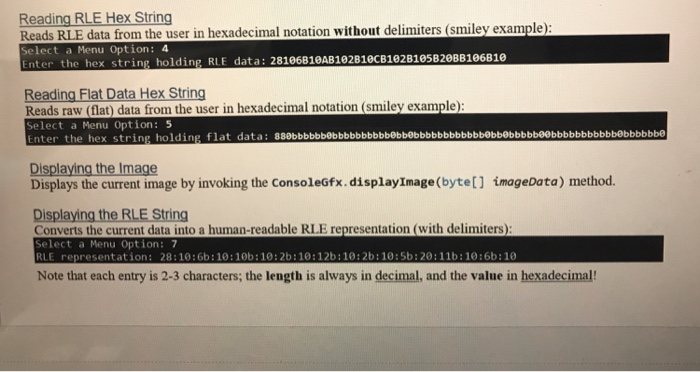This image captures a piece of paper with a horizontal crease running across the lower section from left to right. The paper is filled with detailed information formatted in various sections, each with distinct headers and instructions, typical of a technical document or a user guide.

At the top, the first section header, "Reading RLE Hex String," is prominently underlined and rendered in blue font. Below this header, it is stated that the process "reads RLE data from the user in hexadecimal notation without delimiters". An example, denoted by a parenthetical smiley face, is provided. This section features a black bar that contains two lines of text:
1. "Select a menu option: 4"
2. "Enter the hex string holding RLE data," followed by a lengthy string of letters and numbers approximately 20 characters long.

Moving to the next section, the header "Reading Flat Data Hex String" appears, also underlined and in blue font. This section explains that it "reads raw (flat) data from the user in hexadecimal notation," and similarly displays an example with a smiley face in parentheses. Below this, it instructs the user to:
1. "Select a menu option: 5"
2. "Enter the hex string holding flat data," followed by a much longer string (about 30 to 40 characters) dominated by the digits '8', 'B', and '0'.

The subsequent section is titled "Displaying the Image," with the header underlined and in blue. The text describes the function that "displays the current image by invoking the console GFX," specifically "consoleGFX.display.displayImage(BYTE[] imageData)". Both "consoleGFX" and "BYTE" are highlighted in blue.

Following this, the next section is labeled "Displaying the RLE String," maintaining the underlined and blue font format. This part of the document details how to "convert the current data into a human-readable RLE representation" with delimiters included. A black bar further instructs:
1. "Select a menu option: 7"
2. "RLE representation," showcasing a series of numbers and ratios in the format "28:10:6B:10:10B," extending through another 10 or 12 sets.

At the bottom of the document, a note clarifies that each entry is two to three characters in length. The term "length" is rendered in bold and underlined, noting that it is always presented in decimal. In contrast, the term "value" is highlighted in bold black and underlined, indicating it is displayed in hexadecimal notation. The final line concludes emphatically with an exclamation mark.